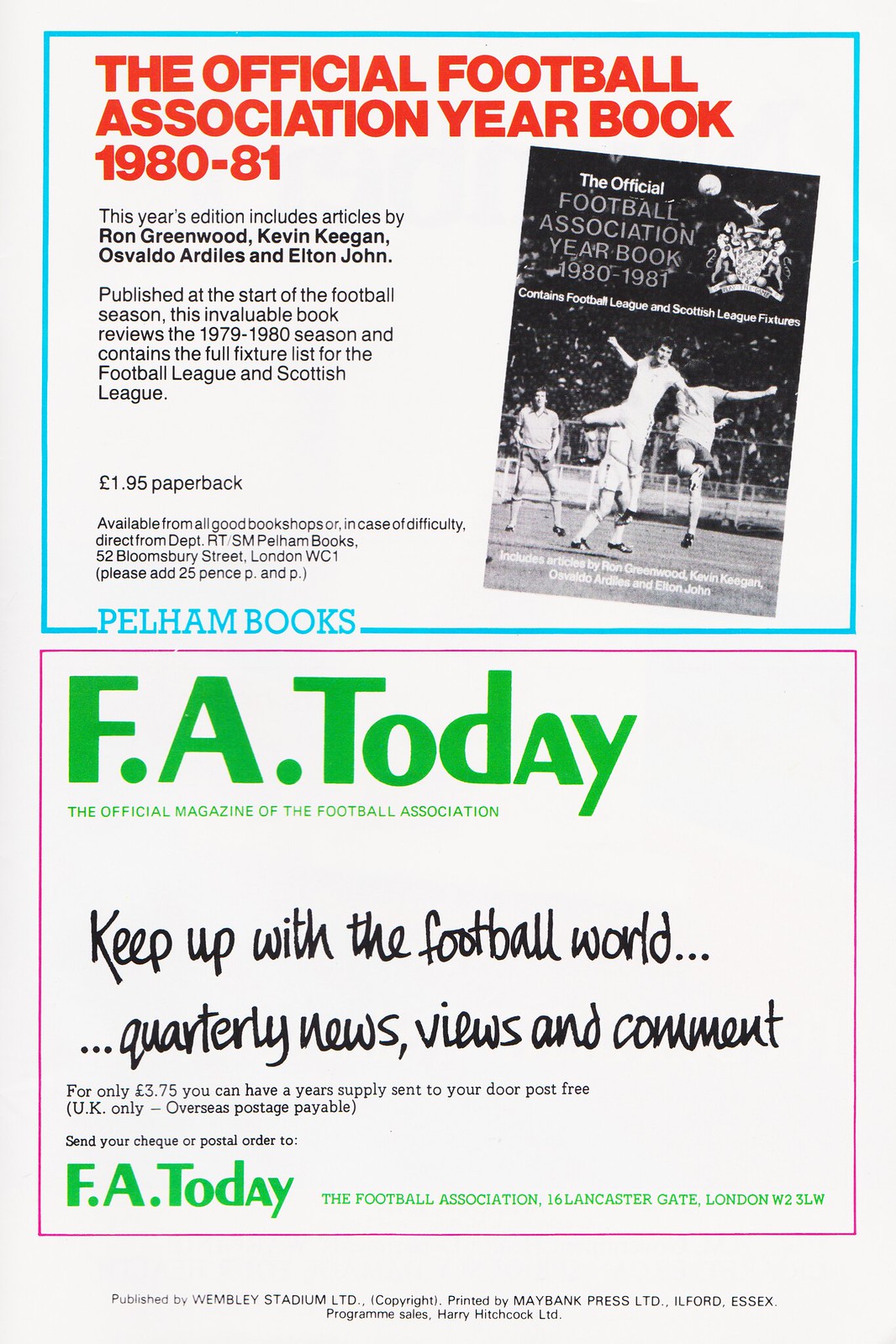This image depicts two vertically stacked advertisements from a football program or magazine. The top advertisement is framed by a turquoise blue border and features red font. It promotes "The Official Football Association Yearbook 1980-81" and includes a black-and-white image of the yearbook, which pictures soccer players in action. The ad details that the yearbook contains articles by prominent figures such as Ron Greenwood, Kevin Keegan, Osvaldo Ardiles, and Elton John. It reviews the 1979-1980 season and provides the full fixture list for the Football League and Scottish League, all for $1.95, published by Pelham Books.

The lower advertisement is set within a pink border, and the green font at the top reads "FA Today." In black font below, it announces "Keep Up With The Football World: Quarterly News, Views, and Comment." This section further notes that FA Today is the official magazine of the Football Association and is priced at $3.75. Both ads include various smaller details to inform and entice the reader.